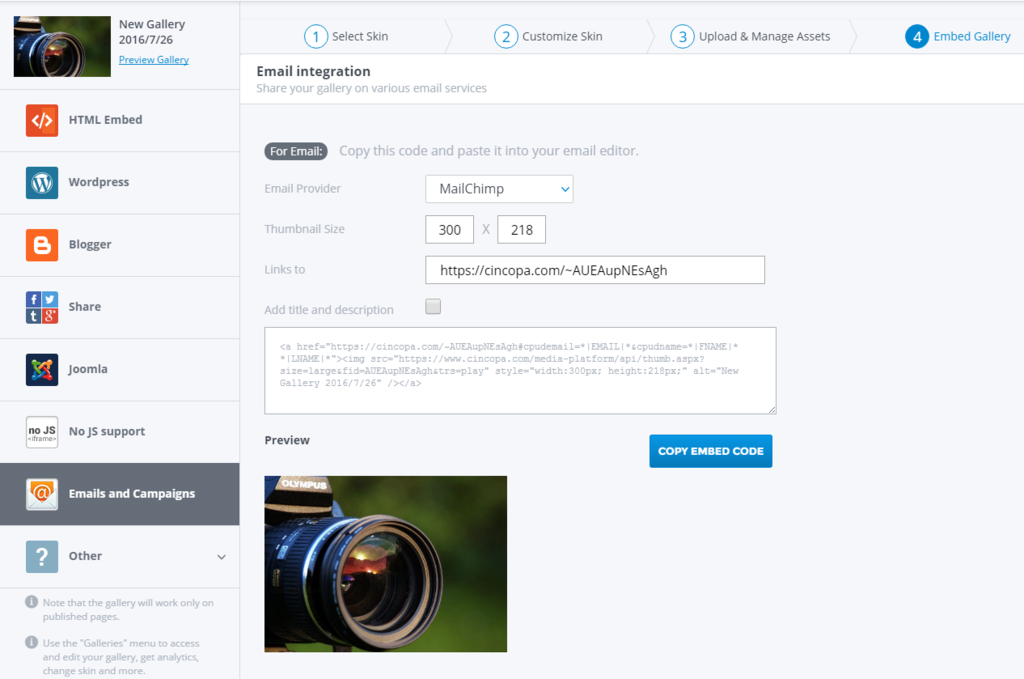This image showcases the setup interface for a photo gallery display, likely geared towards customizing and embedding the gallery into various platforms and email services. 

On the left-hand side, there's a vertical navigation column labeled "New Gallery 2016-726 Preview Gallery," highlighted by a digital camera icon at the top. Below this, several options are listed for embedding the gallery, including HTML, Embed, WordPress, Blogger, Share, Joomla, Node.js Support, and Emails and Campaigns. The "Emails and Campaigns" option is currently selected and highlighted by a gray box.

A note at the bottom of this column states, "Note that the gallery will work only on published pages," followed by instructions to use the gallery's menu to access and edit the gallery, obtain analytics, change the skin, and more.

On the right-hand side, a configuration bar provides options for customization:
1. **Select Skin:** Choose the visual theme for the gallery.
2. **Customize Skin:** Modify the chosen skin to suit specific preferences.
3. **Upload and Manage Assets:** Manage the images and assets for the gallery.

Further down, there's a section titled **"Email Integration,"** which assists in sharing the gallery through various email services. This section includes a gray box with instructions, "For Email: Copy this code and paste it into your email editor." Below this, a drop-down menu currently set to "MailChimp" allows selection of different email providers. Thumbnail dimensions are set to 300 by 218 pixels, linking to https://cincopa.com, and some assigned code is visible.

Finally, there is an option to add a title and description, as well as a blue button labeled "Copy Embed Code" for easy copying and pasting into desired platforms.